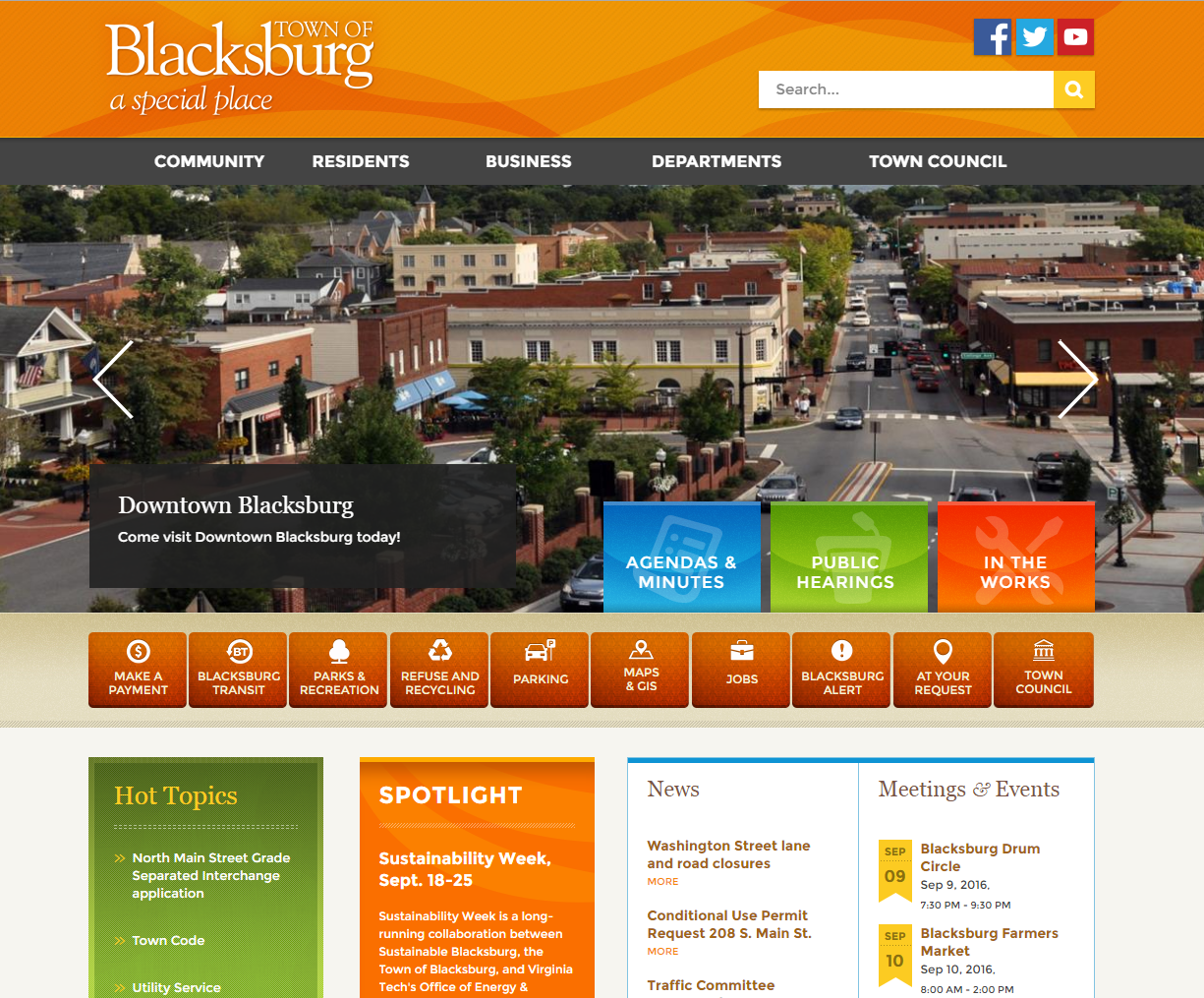At the top of the image, there is an orange banner featuring an abstract pattern consisting of swirls and circles in varying shades of light and dark orange. On the left side of the banner, the word "Blacksburg" is displayed in a white font. Towards the right side of the banner, the words "TOWN OF" are written in smaller capital letters, and at the bottom of the banner, the phrase "A special place" is italicized.

Adjacent to the right of the text, there are three square icons for social media platforms: the Facebook icon, the classic Twitter icon, and the YouTube icon. Below these icons, there is a search area with placeholder text "Search..." in grey lettering, framed by a light grey shadow. To the right of the search bar, there is a yellow box containing a white magnifying glass icon pointing to the left.

A dark grey strip runs below the banner, serving as a menu bar with white text options. The menu includes categories such as "Community," "Residents," "Business," "Departments," and "Town Council."

Below the menu strip is an image depicting a panoramic view of a town, showcasing several brick and concrete buildings along with a roadway populated by several cars in transit. 

At the bottom of the image, there is a black banner with low opacity, making it semi-transparent. In bold white text, the banner reads "Downtown Blacksburg." Beneath this, in smaller white letters, it says "Come visit downtown Blacksburg today!" 

To the right of the banner, three colored squares are displayed: the first is blue with the text "Agendas and Minutes," the second is green with the text "Public Hearings," and the third is orange with the text "In the Works."